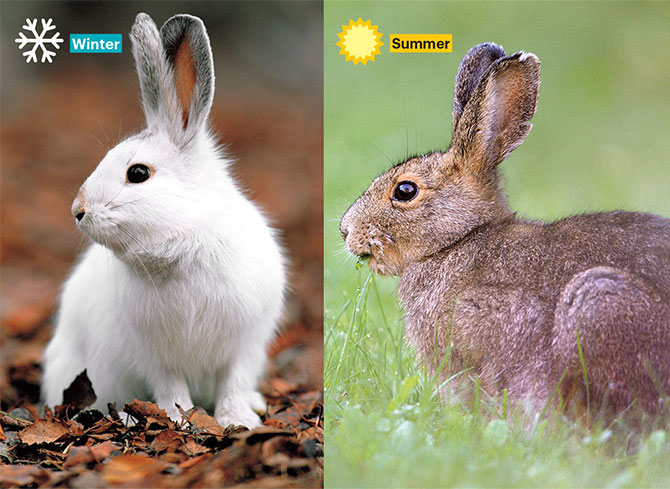The image is a combination of two distinct photographs representing different seasons, titled "Winter" and "Summer". On the left side, labeled "Winter" in white font within a blue box, is a picture of a white rabbit with brown eyes and grayish ears, nestled among brown, reddish, and orange leaves scattered on the ground. A snowflake icon is displayed in the upper left corner of this side. The rabbit is facing towards the left, with its body positioned towards the front of the image. On the right side, labeled "Summer" in black font within a yellow box, a brown bunny with varying shades of brown fur and a whitish nose is depicted. This rabbit is crouching in tall green grass, also facing left, while a sunshine icon occupies the upper left corner of the summer image. The contrasting depictions of the rabbits in their respective seasonal settings highlight the differences in their environments and appear to suggest the passage of time from winter to summer.